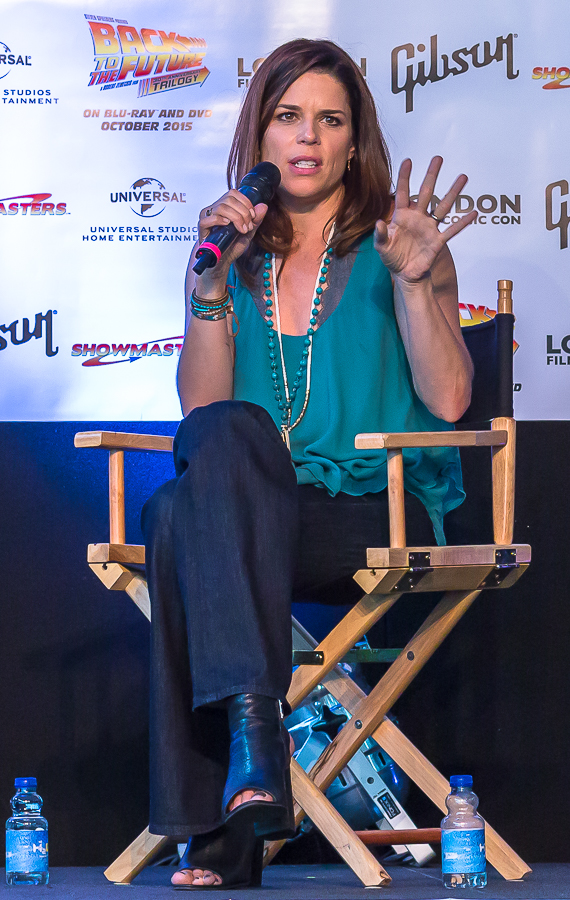A woman is seated on a director's chair in front of a white backdrop adorned with an array of colorful text and logos, including black, red, orange, yellow, and blue elements. Prominently displayed among the various logos is the Universal Studios Home Entertainment globe logo, as well as a promotion for the "Back to the Future Trilogy" on Blu-ray and DVD, slated for release in October 2015. The backdrop features a tile pattern with these graphics scattered throughout. The woman is wearing a green top, accessorized with a green beaded necklace and another silver necklace. She has long brown hair and is dressed in black pants and black shoes. Holding a microphone, she appears to be speaking, with one hand raised in a gesture. At her feet, there are two water bottles on the ground.